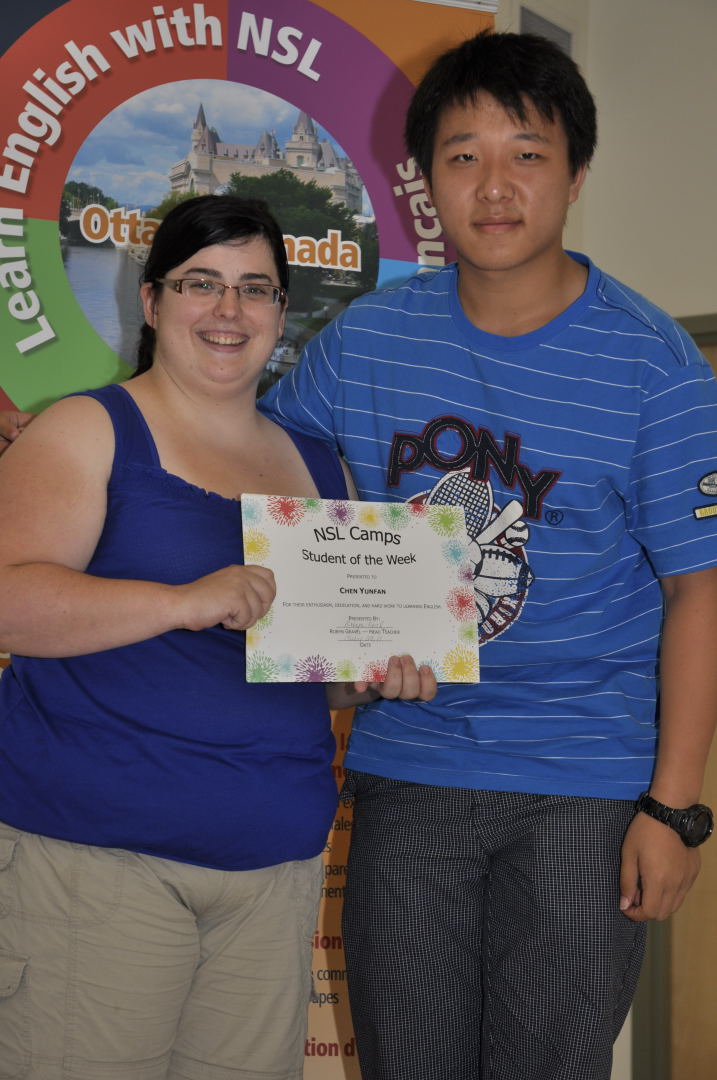In this photograph, we see a smiling woman and an Asian man standing in front of a sign that reads "Learn English with NSL." This sign features an image of a castle and the text "Ottawa, Canada," encircled by a colorful border of green, orange, purple, and blue. The woman, positioned on the left, is wearing a blue strappy top and light brown trousers. She has black hair, wears glasses, and is holding a certificate that reads "NSL Camps Student of the Week" with colorful circles around it. The man on the right, who appears to be the award recipient, has black hair and is dressed in a blue Pony t-shirt with a tennis racket and football logo, paired with checkered trousers. He is wearing a black watch on his wrist and has a small smile while looking at the camera. Both individuals are clearly the focal points, with the woman presenting the certificate to the man, encapsulating a celebratory moment possibly at a school or award ceremony.